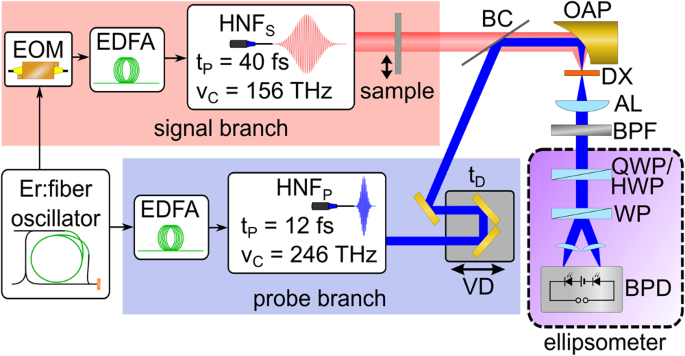The infographic illustrates a complex optical circuit system, combining colorful branches and detailed annotations. In the bottom-left corner, the 'ER Fiber Oscillator' is depicted with a green rolled circle inside a black stand. Arrows emanate from this point: one arrow leads upwards, and another to the right.

The rightward arrow points to the 'Probe Branch,' which includes the labels "EVFA to HNFP or TPE equals 12SS" and "VC equals 246THZ." This branch features a gray square marked 'TV' and a blue line that travels and reflects through a series of reflections, indicating measurements denoted as 'VD,' moving up, left, and diagonally.

Above the Fiber Oscillator, the 'Signal Branch' begins, identified by a pink background. This branch progresses through several stages: 'EOM,' 'EDFA,' and 'HNFS,' with descriptors "TP equals 40FS" and "VC equals 156THZ." The red line from this branch intersects with the blue line, leading to a reflector marked 'OAP.' From here, the blue line transverses various barriers labeled 'DX,' 'AL,' 'BPF,' 'QWP,' 'HWP,' and 'WP,' finally terminating at the 'BPD Ellipsometer.'

Overall, the diagram is vibrant with colors such as pink, blue, and purple, adorned with numerous abbreviations and symbols like EOM, EDFA, HNFS, and QWP, reflecting a sophisticated flow of signals and probes, ultimately converging at the 'Ellipsometer' situated at the bottom right.